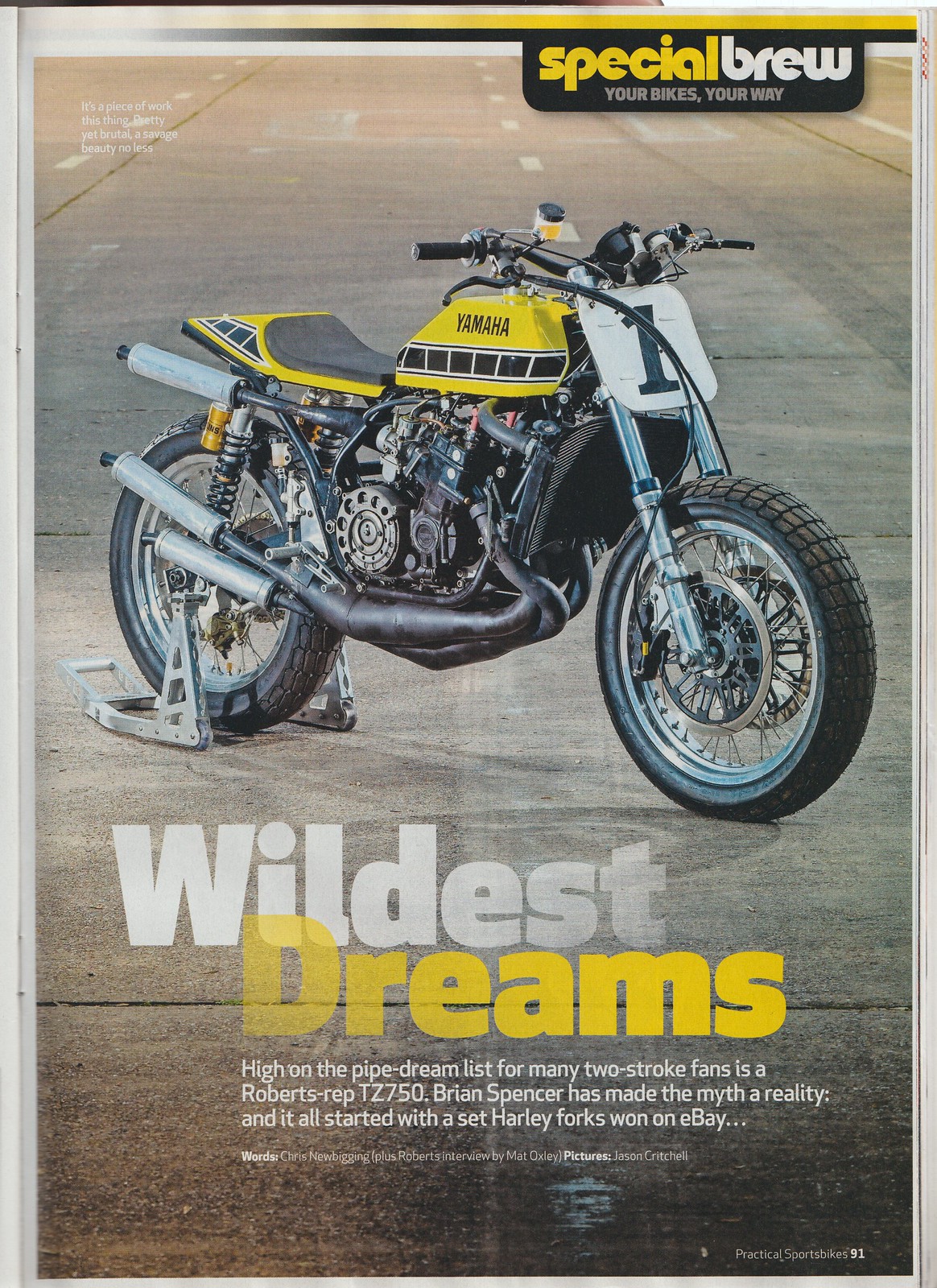This striking advertisement showcases a Yamaha dirt bike, prominently positioned on a plain pavement road marked with white checkered lines. The overall aesthetic is dominated by black and yellow hues, with accompanying white and yellow text that pops against the backdrop. At the top of the poster, the tagline "Special Brew, Your Bike's Your Way" is boldly displayed.

Central to the image is the Yamaha dirt bike itself, characterized by a distinctive combination of gray, black, and yellow. The bike features a yellow-striped tank, reminiscent of a dotted line, and a sleek black leather seat with yellow accents that echo the tank's design. The bike's motor and muffler are finished in black, while the rims are silver, adding a touch of contrast alongside the silver forks. The front of the bike sports a square plate emblazoned with the number one, underscoring its premier status.

Supporting the bike is a metal stand at the back wheels, ensuring stability for the photograph. Below the image of the bike, the bold text "Wildest Dreams" is split between white and yellow, further capturing the viewer's attention. The caption reads, "High on the pipe dream list for many two-stroke fans is the Roberts Rep TZ 750. Brian Spencer has made the myth a reality, and it all started with Set Harley Forks won on eBay." This detailed caption ties together the aspirational theme of the advertisement, celebrating the realization of a cherished dream for bike enthusiasts.